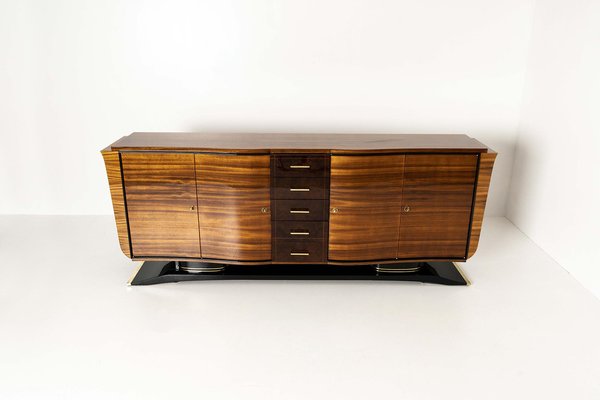This landscape-oriented photograph captures a piece of elegantly crafted wooden furniture, which appears to be a stylized dresser. The surroundings feature pristine white walls and a polished white floor, providing a stark and modern backdrop. The dresser is positioned predominantly on the right side of the image, near the corner where the walls converge. The wooden surface of the dresser exhibits a subtle curvature toward the center, suggesting a blend of artistry and functionality in its design. At the center of the dresser, there are five linear handles, indicating the presence of multiple drawers. The entire piece rests on a sleek, glossy black platform, which adds a striking visual contrast and enhances the overall aesthetic appeal of the setting.